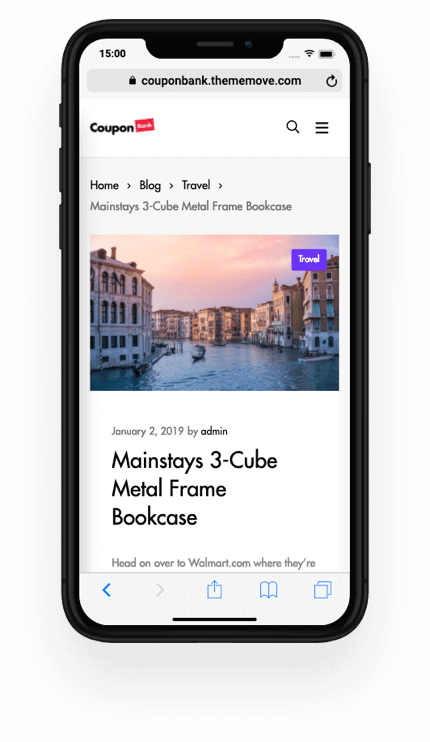A screenshot captures the interface of a mobile site accessed at 15:00 using Wi-Fi, with a fully charged battery. The web address displayed is "couponbankthemeove.com". At the top, there is a header with a hamburger menu on the far right, a central search bar, and the word "Coupon" on the left. This text is presented in black on a white background, accompanied by a small red box labeled "New".

Below the header, there is a gray section featuring a menu with three dropdown options: Home, Blog, and Travel. Under this menu, an advertisement for a "Mainstays Three Cube Metal Frame Bookcase" appears. Further down, a photograph of a Venetian canal is displayed. Below this image, the advertisement for the bookcase is repeated, mentioning that it is available at Walmart.com.